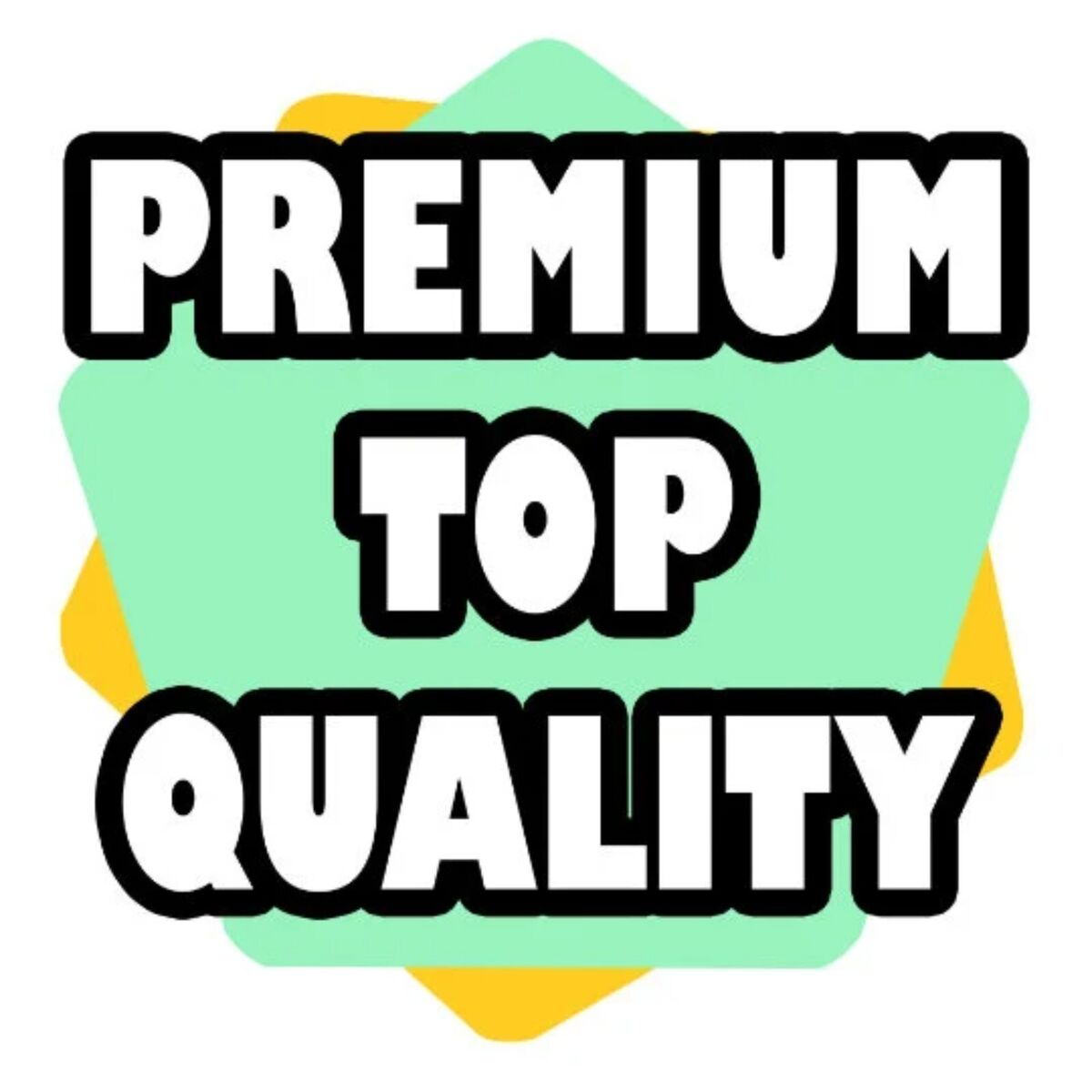The image features bold, chunky, white letters that read "Premium Top Quality" in a 1990s-style font with rounded edges. These letters have a thick black outline that spills out around them in all directions, creating a clustered effect where the black shadows merge together. The background consists of a large turquoise mint green pentagon shape, layered over a similarly sized yellow pentagon. The green pentagon appears to be rotated such that a point sticks out from the top, while the yellow pentagon underneath it is slightly visible, extending points out from the sides and bottom. The entire arrangement is set against a white backdrop, making the colors and the text stand out prominently.